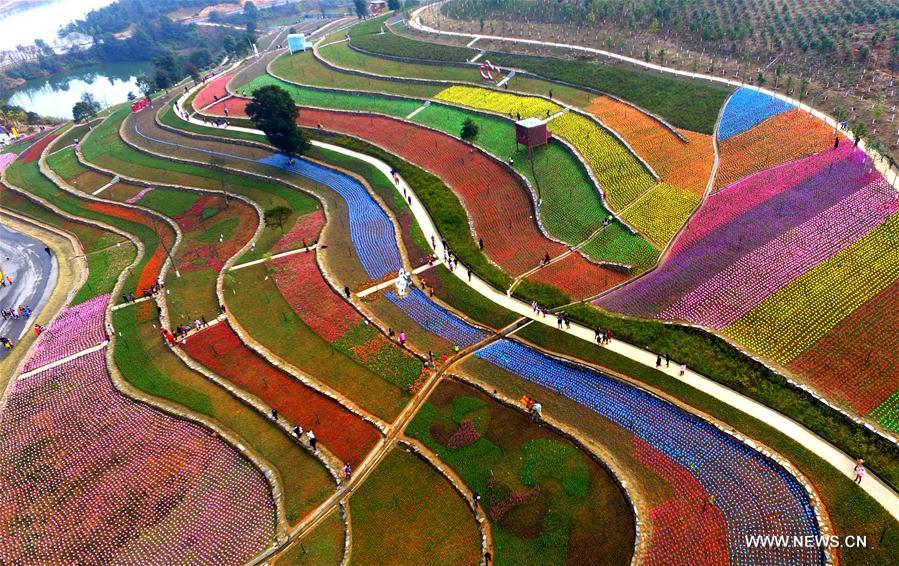This aerial photograph, marked with www.news.cn at the bottom right; depicts a mesmerizing, multicolored landscape composed of curvilinear and segmented agricultural fields. Each section, resembling a tapestry, is planted with various vividly colored flowers and plants, creating bands of green, pink, red, orange, yellow, blue, and purple. A prominent white curved walkway runs centrally through the image, along which people are strolling, intersecting with narrower brown pathways. The lower right section features a vibrant array of colors, while the upper regions depict less vivid agricultural land and small bluffs adorned with trees and shrubs. To the far right, rows of trees can be seen, and in the distant background lies a small body of water, surrounded by greenery. This harmonious blend of nature's colors and human activity provides a striking and intricate view of cultivated beauty.